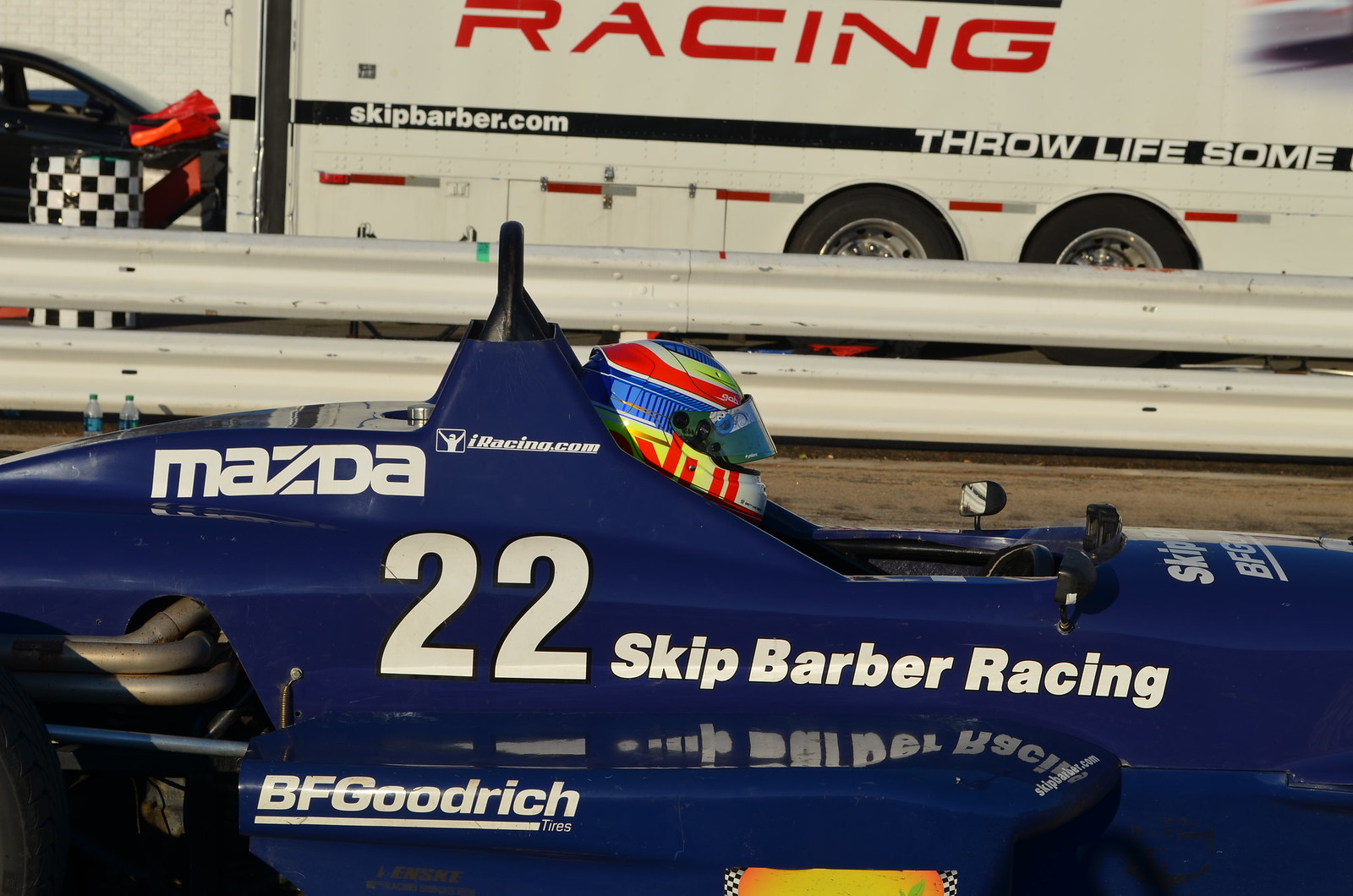This image captures a side view of a sleek, navy blue race car with an open cockpit, showcasing a single driver. The driver's helmet, adorned with vibrant red, blue, neon yellow, and white stripes, features a partially open, tinted visor. The race car prominently displays multiple lines of white text on its side, reading top to bottom: "Mazda," "iRacing.com," the number "22," "Skip Barber Racing," and "BFGoodrich Tires." In the background, a white metal road railing separates the car from a large white trailer, which bears the word "Racing" in bold red letters. The trailer also features a black banner with the text "SkipBarber.com" and "Throw Lifesome" running from front to back. Scattered on the ground next to the guardrail are two water bottles. To the left of the scene, a black car and a monochrome stack of tires add to the dynamic background elements.